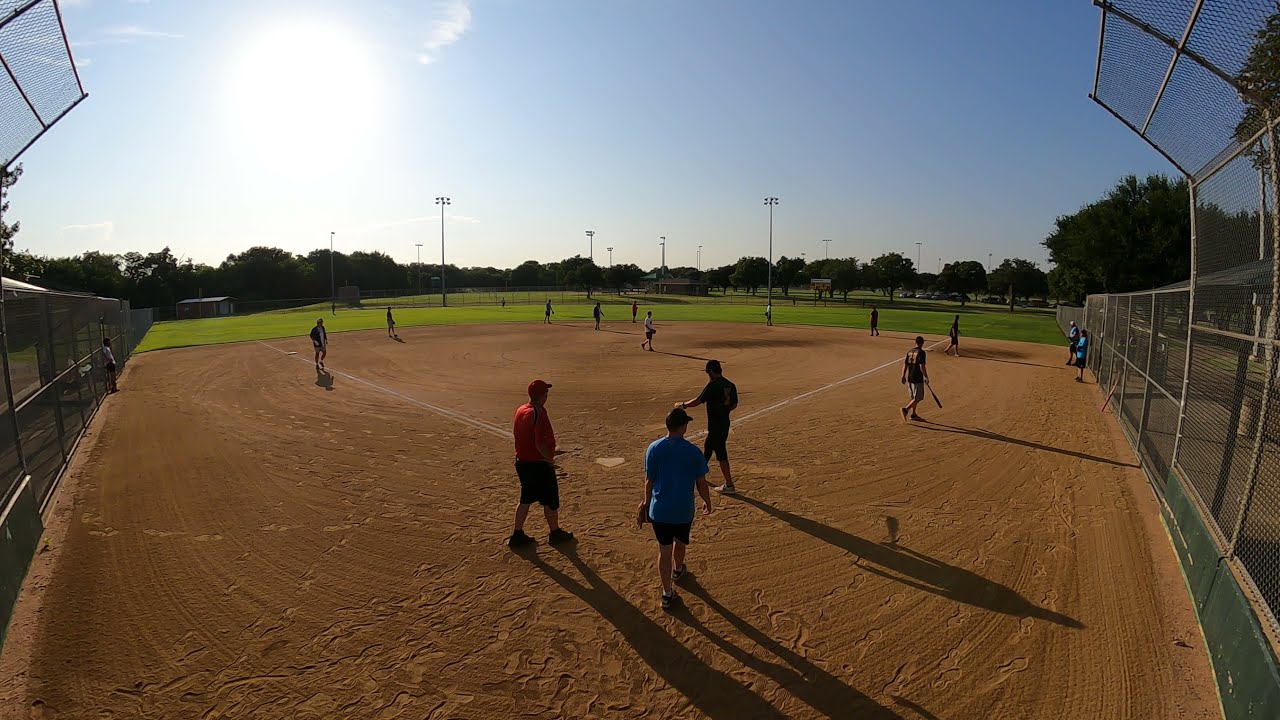This image captures an overhead view of an outdoor baseball field during the daytime. The sky is a gradient of dark to light blue with a few thin white clouds and the bright sun visible. The field is divided into a red clay infield with white lines marking the bases, which are partially covered in dirt. Scattered across the field are multiple individuals, some in casual attire, suggesting this might be a recreational game, possibly in a men’s league. A player in a blue shirt and another possibly serving as an umpire in a red shirt are notable among the participants. The entire area is enclosed by fencing, which is particularly tall near the batter's box. The outfield features closely cut green grass, and in the distance, trees frame the scene. There is also a building resembling a shed or garage in the far distance. Numerous light poles are positioned around the field, indicating the area is well-equipped for night games. The photo seems to have been taken from a slightly elevated position, perhaps by a drone or from a high vantage point, giving a comprehensive view of the field.